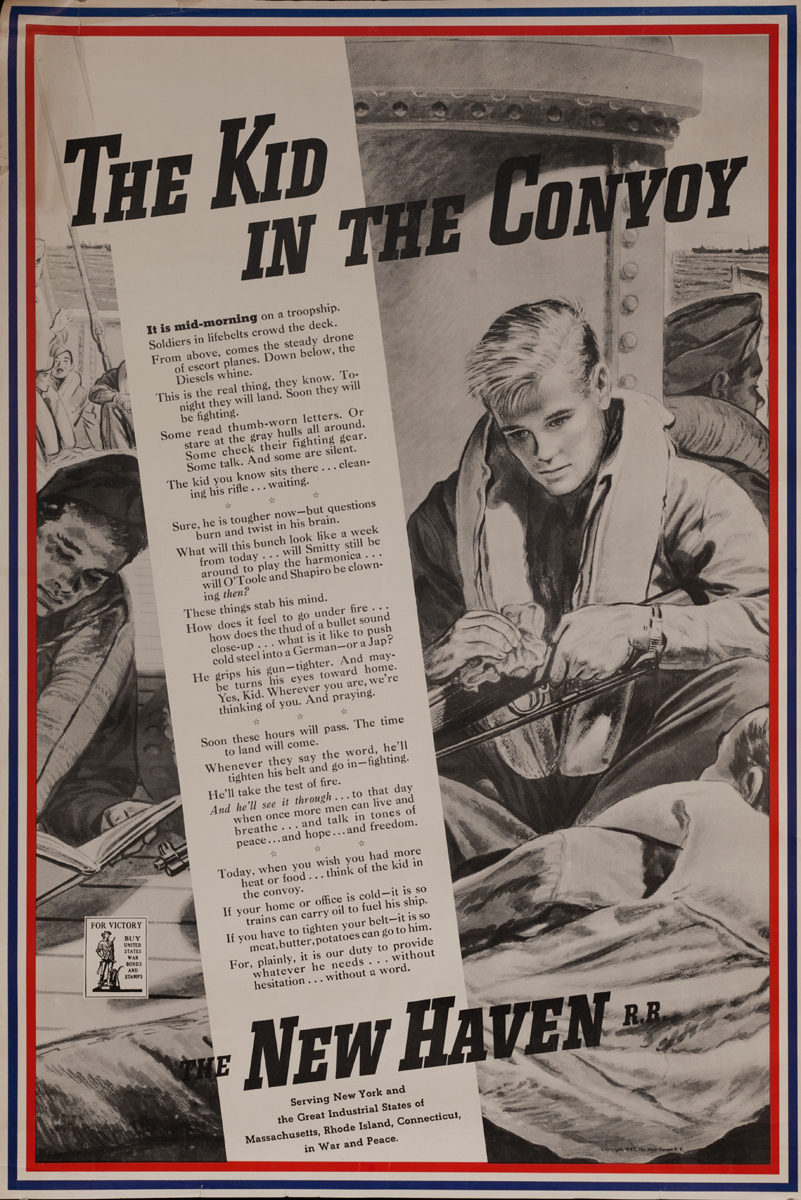This image is a detailed photograph of a vintage magazine page, capturing a hand-drawn illustration of military men during their downtime. The scene is bustling with soldiers in various relaxed poses: some are engrossed in reading books, one is meticulously cleaning his rifle, and others are simply lounging about, embodying a rare moment of reprieve. Superimposed diagonally across this evocative drawing is a poem titled "The Kid in the Convoy." The verses evoke the tense atmosphere of mid-morning on a troop ship, describing soldiers crowded on deck with their lifebelts, the relentless drone of escort planes overhead, and the persistent whine of diesels below. The poem paints a vivid picture of wartime reality and is a poignant reminder of the era. At the bottom of the page, a note indicates that this piece originates from the great industrial states of New York, Massachusetts, Rhode Island, and Connecticut, highlighting their contributions in both war and peace.